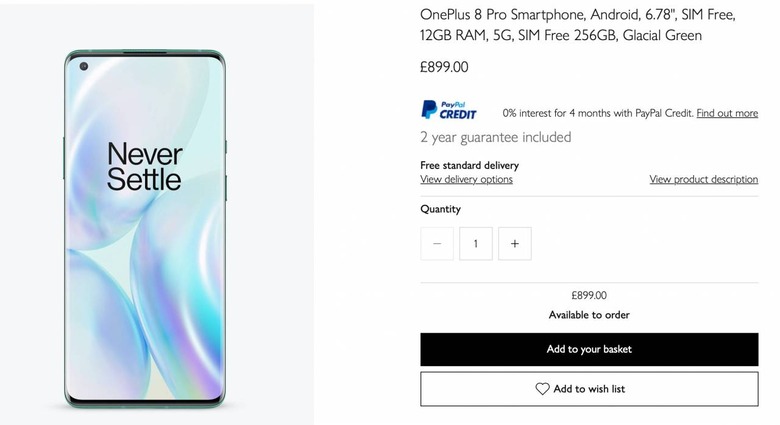In the image, positioned on the far left side, is the front view of a cell phone displaying swirled colors along with the text "Never Settle" on the screen. To the right of the phone, there are product details stating: "OnePlus 8 Pro Smartphone, Android, 6.78 inches, SIM-free, 12GB RAM, 5G, 256GB, Glacial Green, £899.00." Just below this, the PayPal logo is visible with a note that reads: "PayPal Credit, 0% interest for 4 months with PayPal Credit." There is a hyperlink labeled "Find Out More." Further down, it mentions a "2-Year Guarantee Included" and "Free Standard Delivery", followed by another hyperlink titled "View Delivery Options." Adjacent to this is a hyperlink "View Product Description." Beneath these links is the word "Quantity" with a control panel featuring a minus sign, the number 1, and a plus sign for adjusting the quantity. Below this section, the price is reiterated as "£899.00" along with the status "Available to Order." At the bottom, there is a prominent black rectangle with white text reading "Add to Your Basket" and a white rectangle with a black border containing a heart icon and the text "Add to Wishlist" in black font.